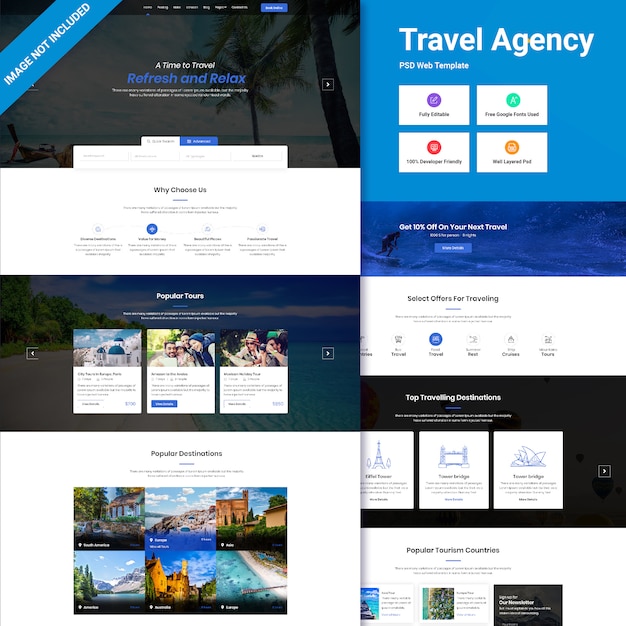**Detailed Image Description:**

The image depicts a square advertisement designed as a web page layout for a travel agency. The ad is divided into two main columns, with the left column being slightly wider than the right one. The overall color scheme transitions from whites to various shades of blue and black.

**Left Column:** 
- **Header:** At the top corner, a vibrant banner reads "Refresh and Relax: A Time to Travel."
- **Section 1:** Below the header, a box titled "Why Choose Us" is displayed, featuring pertinent icons and text to emphasize the agency's advantages.
- **Section 2:** Following is "Popular Tours," which includes three white text boxes, each paired with a photograph and descriptive text about different tour packages.
- **Section 3:** Beneath the popular tours, the phrase "Popular Destinations" introduces a grid displaying six square photographs, representing various appealing travel destinations.

**Right Column:** 
- **Top Section:** The top right portion showcases the title "Travel Agency PSD Web Template" set against a blue background with four white boxes.
- **Middle Section:** Below this, an eye-catching image of a man surfing is visible, accompanied by the text "Get 10% off on your next travel."
- **Lower Section:** Further down, there is a section labeled "Select Offers for Traveling," followed by another section titled "Top Traveling Destinations."
- **Bottom Section:** At the very bottom, smaller text reads "Popular Tourism Countries."

The image is rich with colors, diverse visuals, and informative icons, making it an engaging and comprehensive advertisement for a travel agency.